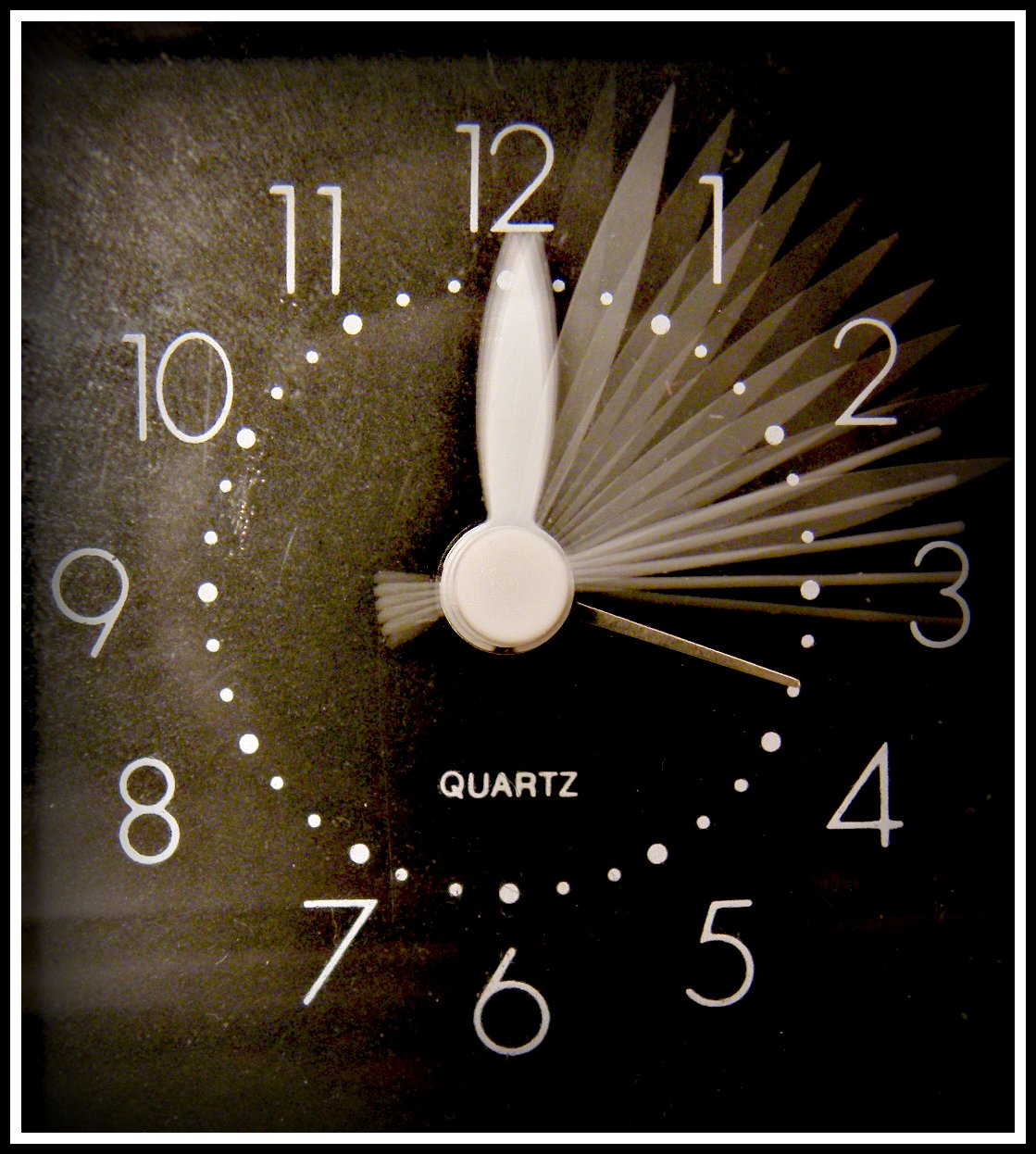This is a long-exposure photograph of what appears to be an old, rectangular analog alarm clock with a worn black face. The clock has both white and silver hands, with the hour hand pointing at 12 and the minute hand pointing near 3, creating an artistic effect through the long exposure which shows the movement of the hands. The alarm is set at 3:45 a.m. with a small golden stick. The clock face shows signs of age, with parts appearing white due to wear, especially on the left side. Surrounding the clock face is a black border with an inner white border. The clock has bold white numbers from 1 to 12 arranged in a circular fashion, with smaller dots corresponding to each hour and even smaller dots between the numbers. There is a faded logo, "Quads," just below the center of the clock face. The design on the clock includes a fan-like white pattern extending from 12 to 3. This time-lapse photograph captures the essence of the old, worn clock, highlighting its detailed features and the passage of time.